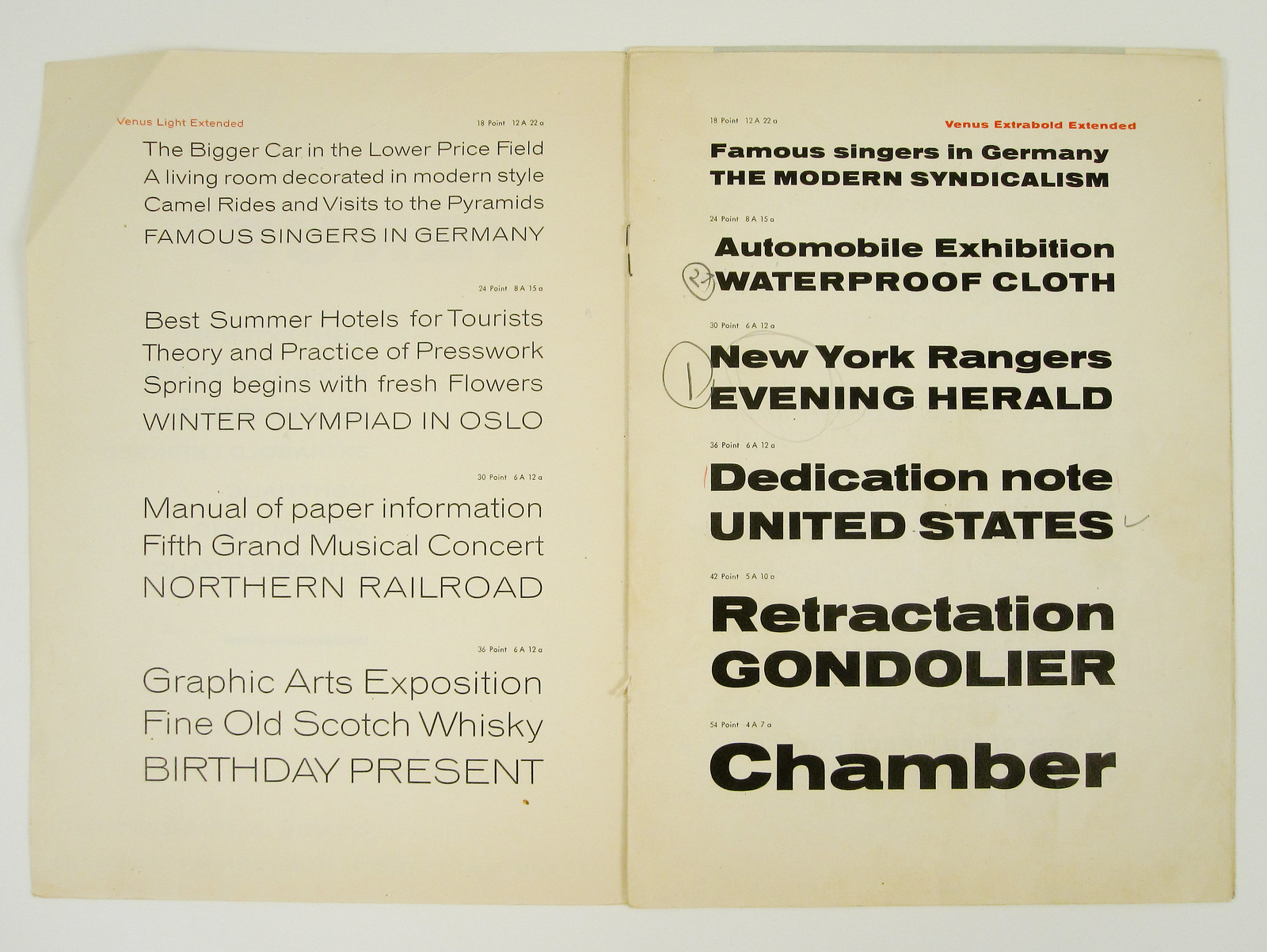The image depicts an open booklet laid flat with its sides spread out, revealing aged, off-white pages. The book is held together by visible staples at the top and bottom, and the upper left corner of the left page is creased from being folded down. The text is primarily in black print, with sporadic red text. The paper appears yellowed and brownish, adding a vintage feel. The left page includes various phrases in red and black text, such as "Venus Light Extended," and "famous singers in Germany," alongside other seemingly random lines like "the bigger car in lower price field" and "theory and practice of press work." The right page features prominently bold, black text: "Venus Extra Bold Extended," "famous singers in Germany," "the modern syndicalism," "automobile exhibition," "waterproof clothes," "New York Rangers Evening Herald," "dedication note," "United States," "retraction," "gondolier," and "chamber." Both pages are filled with an eclectic array of topics, indicating possible snippets of various advertisements, articles, or headlines.